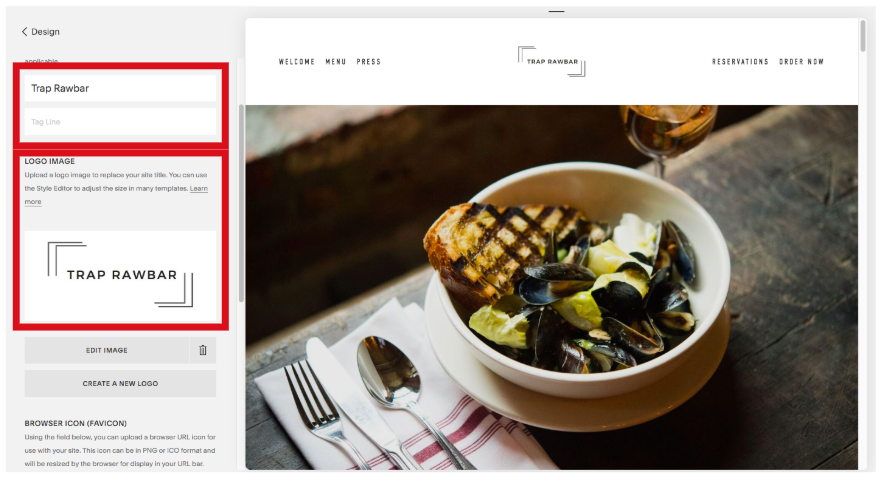Sure! Here's the cleaned-up and detailed descriptive caption for the image:

---

The web page design layout features a gray sidebar on the left-hand side and an equally light gray top bar. On the top left edge, "DESIGN" is prominently displayed in black font alongside a "<" (less than) sign to its left. Adjacent to this is a section highlighted by a thick, red Sharpie-drawn horizontal rectangle. Inside this rectangle, in the upper white space, the words "TRAP RAW BAR" are printed in bold black letters, while the second white space remains blank.

Below, a vertical rectangle with a red border encloses the text "LOGO IMAGE" in all capitalized black font. Beneath this, there's small, challenging-to-read text. Further down on a white background, the title "TRAP RAW BAR" is capitalized and in black font. This is all contained within the second red-outlined section.

Directly beneath this, there is an "EDIT IMAGE" button on a gray background and a "CREATE A NEW LOGO" button underneath it. At the very bottom, the text "BROWSER ICON (FAVICON)" appears, although it is too small to read clearly.

This entire left section occupies about one-third of the image. The right two-thirds begin with a white rectangular area at the top, featuring "WELCOME", "MENU", and "PRESS" in black capital letters, aligned horizontally. Central to this section is the "TRAP RAW BAR" title. To the right, "RESERVATIONS" and "ORDER NOW" are also displayed prominently.

The image showcases a slightly overhead view of a rustic table setting. Centrally placed is a bowl, likely containing oysters and possibly a piece of fish, resting on a plate. A napkin to the left holds a fork, knife, and spoon, although their handles extend beyond the bottom left corner of the photo. Also visible is a partially cut-off wine glass to the right of the bowl. The entire arrangement sits atop a rustic brown wooden table, giving a cozy and inviting dining ambiance.